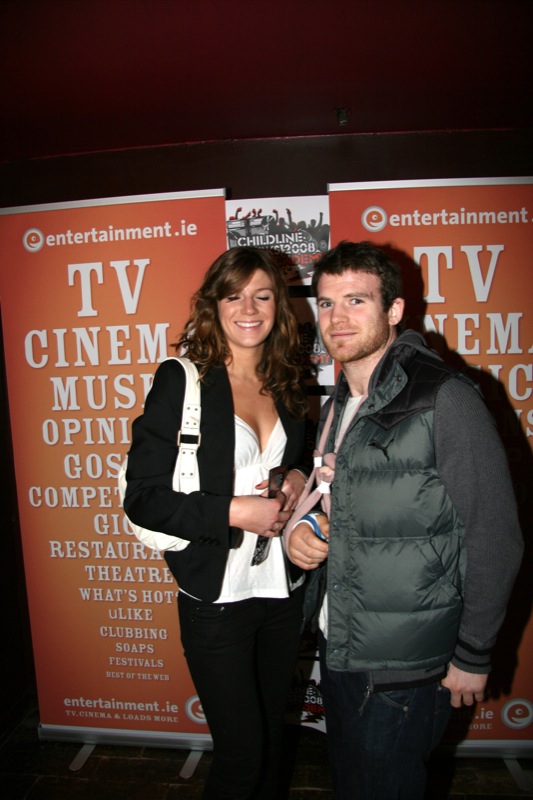This photograph captures a young couple standing in front of a promotional banner for "Entertainment.ie." The image, vertically aligned with black borders at the top and bottom, appears to be set in a room with dark red walls. On the left stands a woman with long wavy brown hair, smiling with her eyes closed. She is dressed in black pants, a low-cut white shirt, a black jacket, and has a white purse over her right shoulder. Beside her on the right, a man with short brown hair and a thin beard is wearing a puffy black jacket over a black long-sleeve top, paired with dark jeans. His right arm is in a blue cast, supported by a pink sling. The banner behind them features large white print on an orange background at the top, and reads "Entertainment.ie." It lists various entertainment categories including TV, cinema, music, theater, gossip, competitions, what's hot, clubbing, soaps, festivals, and best of the web. Both individuals, who are likely not celebrities, appear to be enjoying a moment together, making the scene feel candid and relatable.